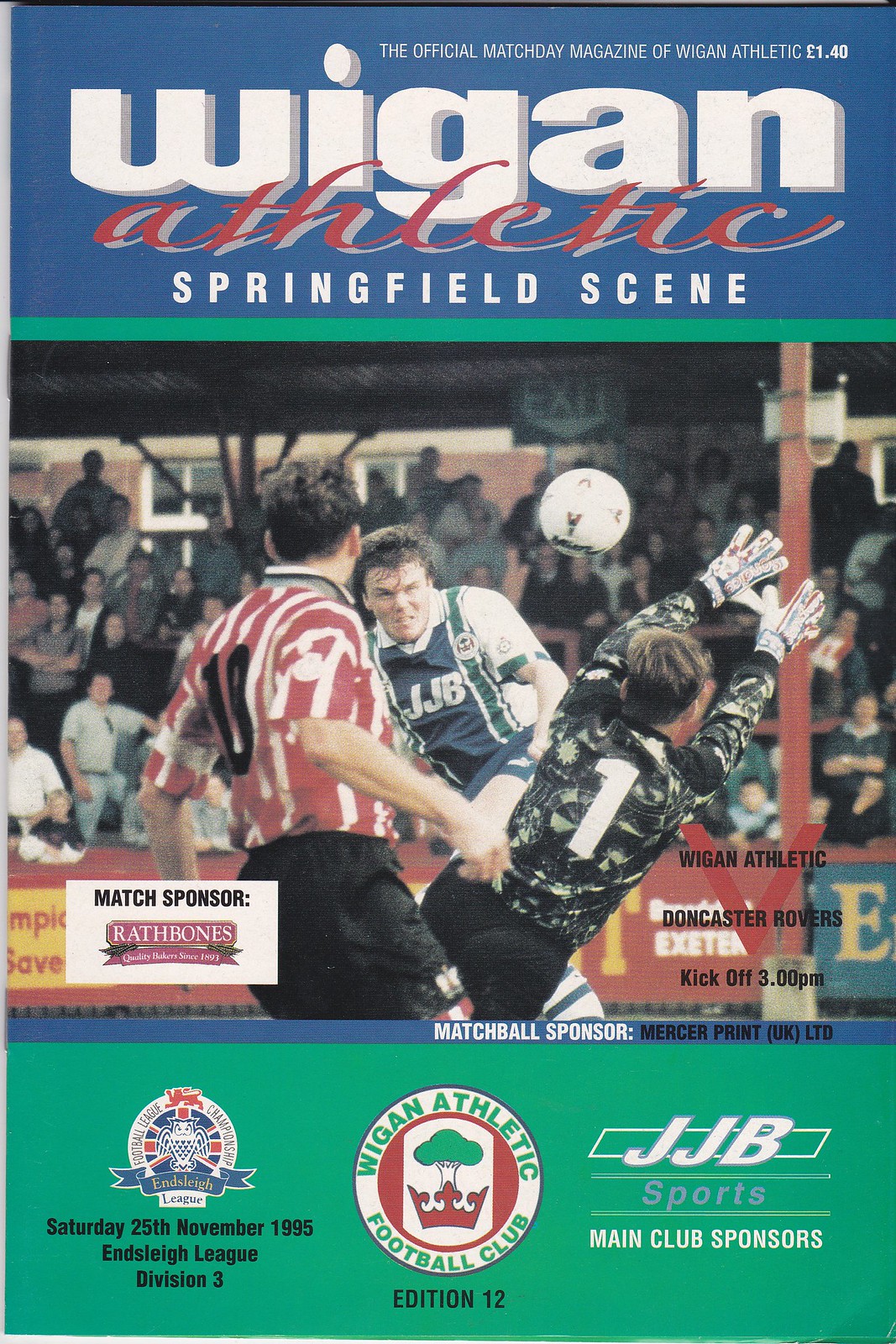The cover of the official Match Day magazine of Wigan Athletic from November 25, 1995, features a vibrant soccer scene. At the top of the cover, a blue banner displays white text that reads, "Wigan Athletic Springfield Scene," with "Wigan" in bold type and "Athletic" below in a red cursive font. A green border separates the title from the main image. The central photograph captures an intense moment on the field: a player in a blue and green striped jersey with white shoulder panels and green sleeve ends has just kicked the ball. To his right, a goaltender in a camel-colored jersey with the number one and distinctive black hair with yellow highlights is leaping to block the ball with outstretched arms. Another player in a red and white striped jersey with black shorts stands behind the goalie, likely a teammate. Spectators fill the stands in the background, adding to the lively atmosphere. Below the main image, text details the match information: "Wigan Athletic vs. Doncaster Rovers, kickoff 3 p.m." and "Match Sponsor Rathbones." A thin blue border at the bottom lists "Match Ball Sponsor Mercer Print." The very bottom of the cover, highlighted in green, features a circular club badge with a crown and tree design, stating, "Wigan Athletic Football Club Edition 12," with additional text indicating "Saturday 25th November 1995, N. Sleigh, League Division 3," and sponsorship information from JJB Sports.